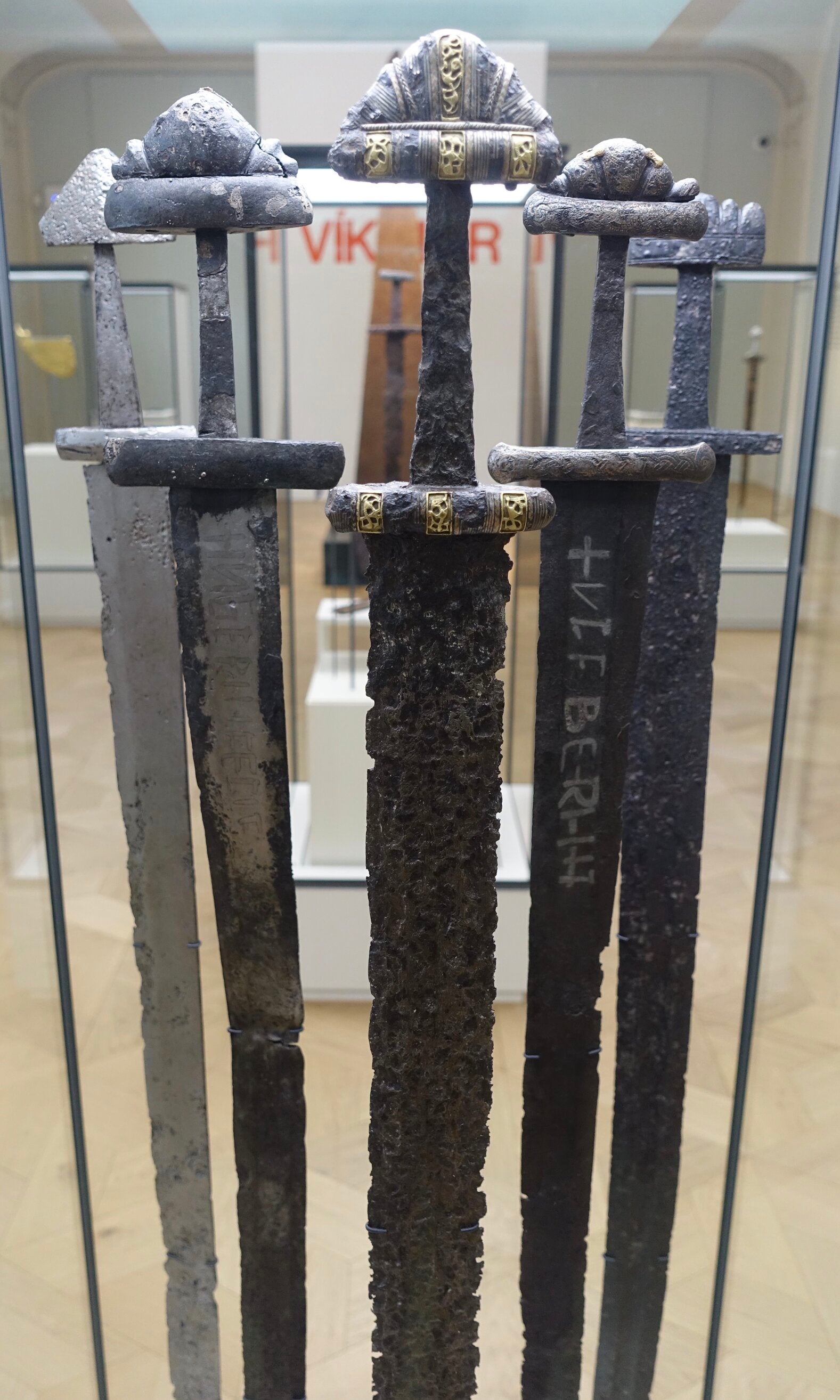In this photograph, we see a close-up shot of five ancient swords showcased in a museum display. The swords are mounted securely, all pointing downwards, which highlights their ornate handles and rusted, jagged blades. The central sword, adorned in black and gold, is flanked on each side by two other swords: to its immediate left, a dark grey sword with lighter grey accents, and further back, a silver sword. To its immediate right is a brass-colored sword with various inscriptions that seem to be in an ancient language, and behind it, a rough-textured, blue-grey sword completes the display. Each sword features unique, intricately detailed designs on their handles, emphasizing their historical craftsmanship. The background, though slightly blurry, reveals the letters "V-I-K" and "R," indicating potential labeling or signage, and other museum exhibition cases, suggesting a larger collection beyond this focused display. These ancient metallic swords stand out prominently against the subdued backdrop, offering a glimpse into their historical significance and ornate beauty.